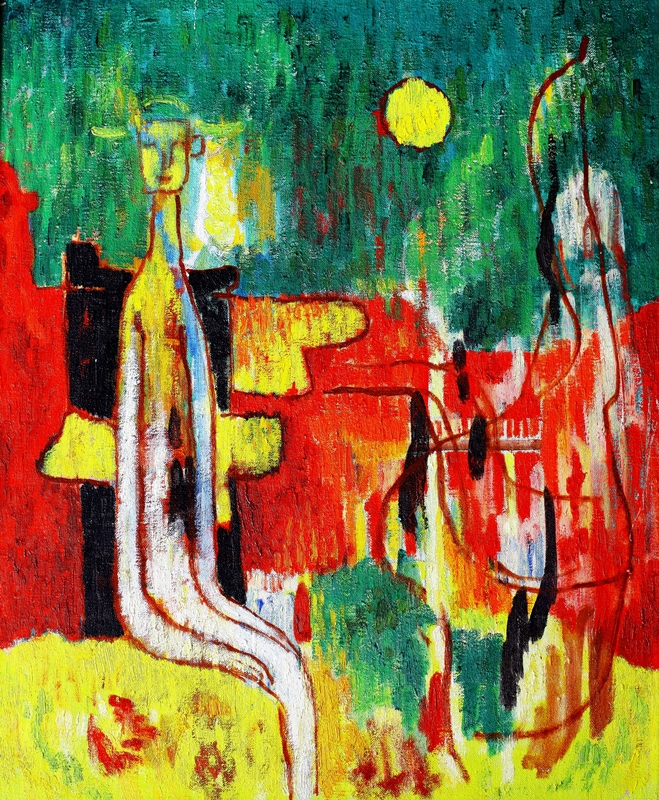This image is a vibrant, abstract painting rendered in various crayon colors, evoking a sense of chaotic energy. The top portion features a greenish-blue sky with a vivid yellow sun slightly off-center to the right, resembling a lemon. Dominating the central part of the artwork is a wavy expanse of red and orange hues, possibly representing flames or a building engulfed in fire. In the midst of this intense scene, a tall, thin man with an elongated neck, arms, and torso is depicted sitting, possibly on a hay bale or a black chair. He is shown in white, staring directly at the viewer, creating a focal point amidst the chaos. The lower section is predominantly yellow with some green, and scattered red footprints suggest a burning or heated surface. To the right, faint outlines appear, which might represent the shape of a woman or perhaps wisps of smoke. The overall scene is a blend of surreal elements and vivid colors, capturing a sense of dynamic tension and abstract beauty.